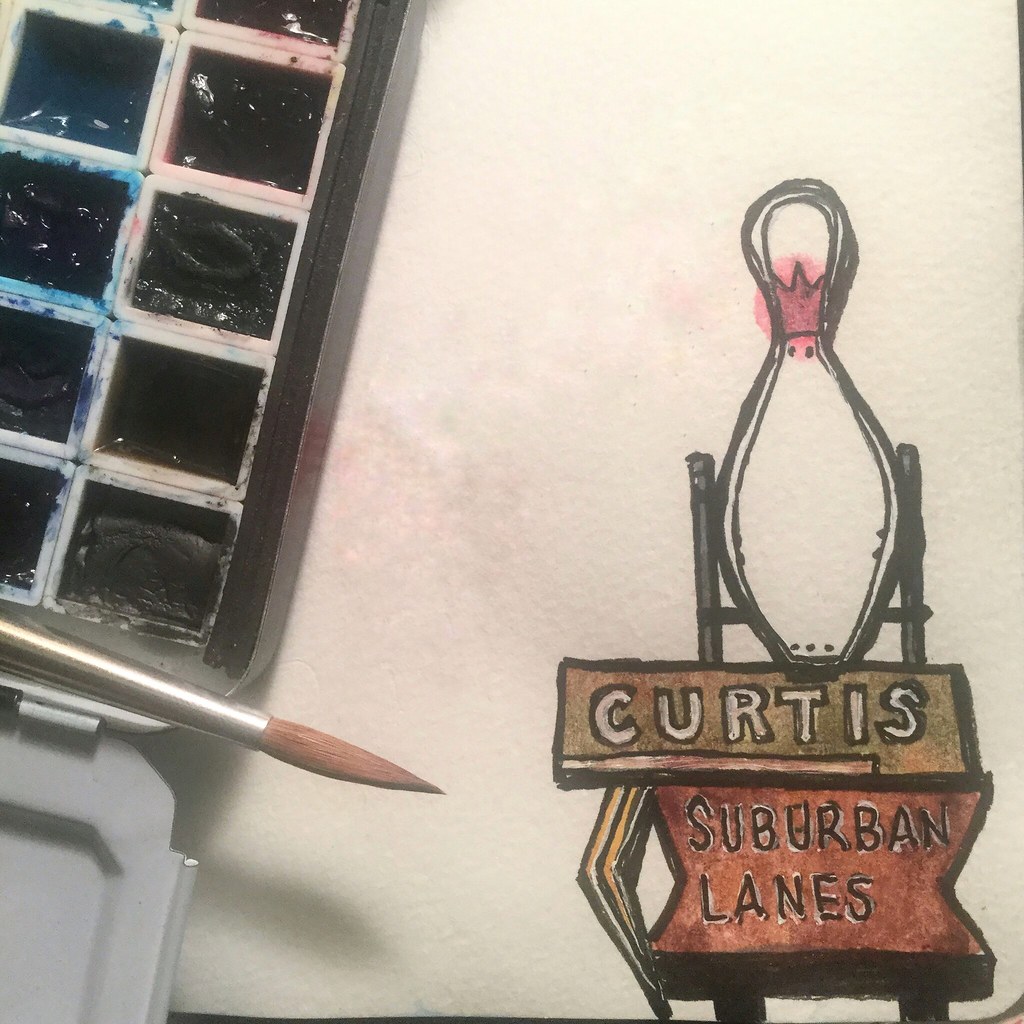In this detailed close-up view, an artist is diligently at work, capturing every nuance on a white canvas or thick watercolor paper positioned on the right side of the image. On the left side, a palette with various shades of black paint is visible, with an artist's pointed brush resting on the edge of this open tray. The hinged lid of the tray can be seen to the far left of the photo. The artist's current project appears to depict an outdoor sign featuring a bowling pin at the top, beneath which the text "Curtis" is written, followed by "Suburban Lanes" in muted beige and red watercolor hues. The bowling pin itself is rendered in white with a distinctive red band near the top. Soft lighting illuminates the room, casting a subtle shadow under the artist's active brush, highlighting both the precision of the painter’s strokes and the intricate details of the artwork.